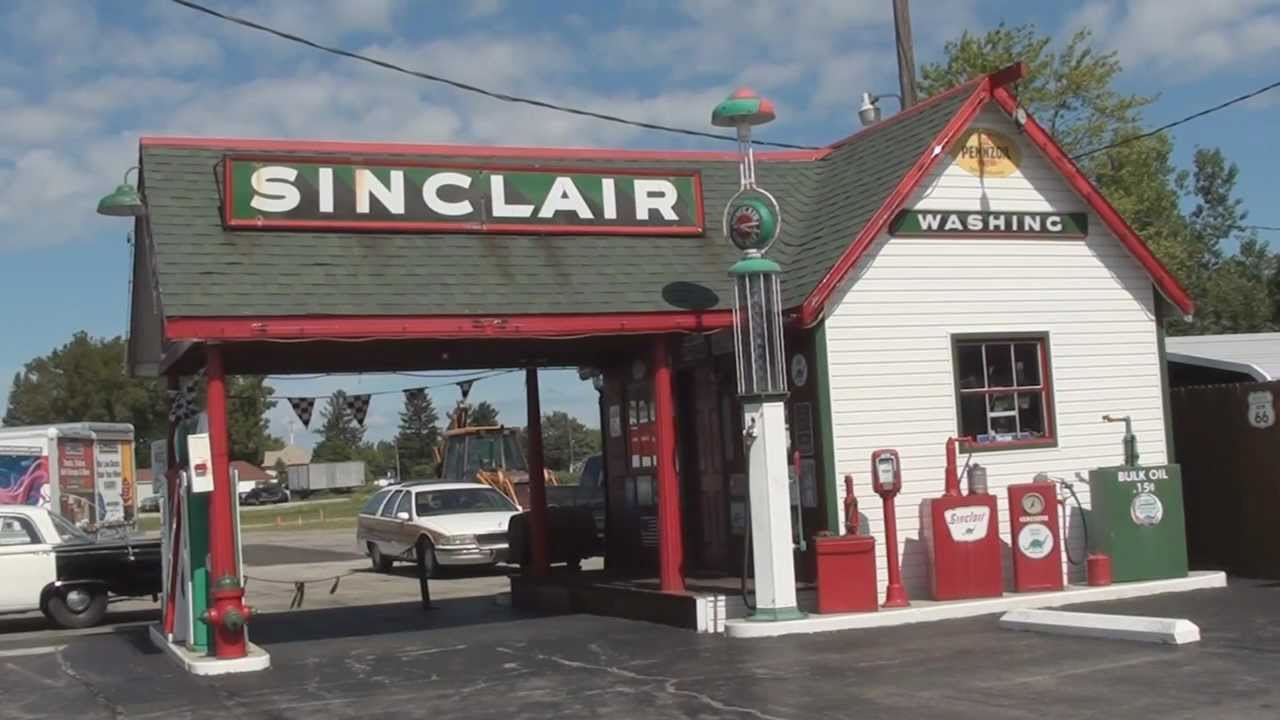This image depicts a meticulously restored vintage gas station, primarily painted white with prominent dark green and red accents. The station prominently features a large overhang supported by two pillars, beneath which two classic gas pumps and a fire hydrant are situated. Emblazoned on a red box atop the overhang is the word "Sinclair" in bold white letters. The main building to the right is constructed with white walls and a triangular roof, beneath which a small, hard-to-read yellow sign is mounted, as well as a rectangular sign that says "Washing." A notable feature is an antique round-faced clock positioned near the building. Visible to the right are various oil canisters and pumps, including a green box labeled "Bulk Oil 15 cents," adding to the nostalgic ambiance. Parked against the building are several vintage cars, including a station wagon, set against a backdrop of puffy white clouds and green trees. The overall appearance, along with checkered racing flags and a roped-off garage area, suggests this exhibit might serve as a historical display rather than a functioning gas station.